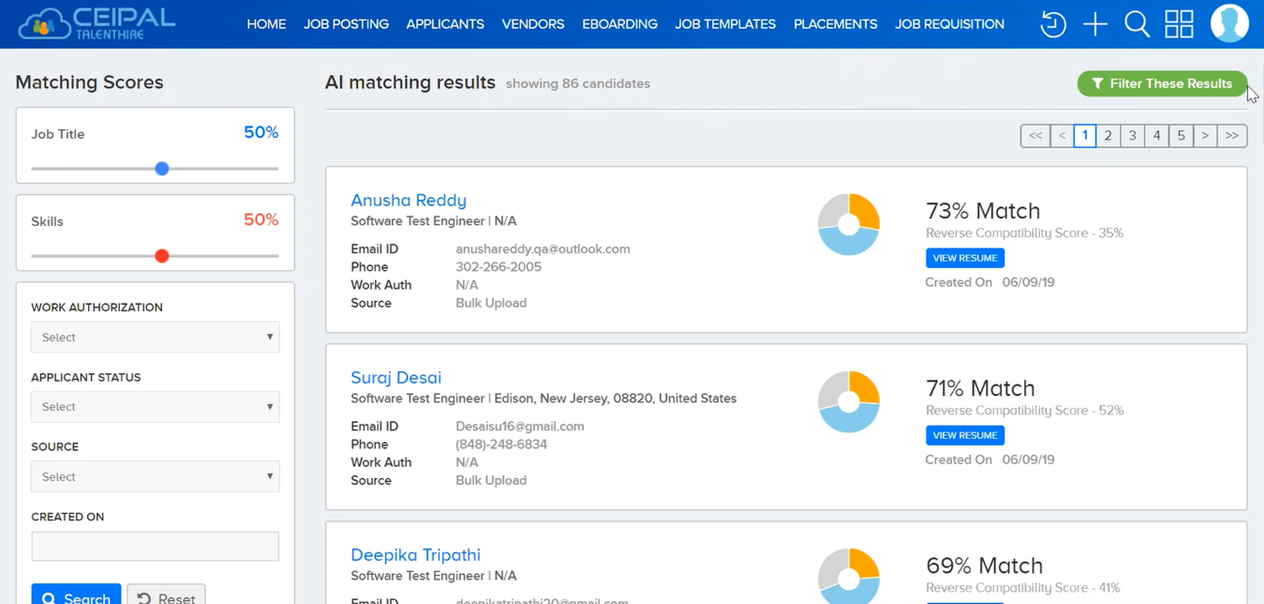The image features a detailed webpage interface for CEIPAL TalentHire, a talent acquisition platform. Dominating the top section of the page is a white cloud outline with the name "CEIPAL TalentHire" displayed in soft gray font against a light blue background. 

Positioned at the very top are clickable options in white, enhancing the site's navigation. These navigation tabs include: Home, Job Postings, Applications, Vendors, eBoarding, Job Templates, Placements, and Job Requisition.

On the right-hand side, a series of distinctive white icons are neatly arranged. These include:
1. An arrow enclosed within a circle bearing a backward L shape.
2. A plus sign.
3. A magnifying glass.
4. Four smaller squares forming a larger square.
5. The silhouette of a person within a white circle.

A highlighted section in a green bubble prominently mentions that AI matching results have identified 86 candidates. This segment also offers filtering options for refining these results.